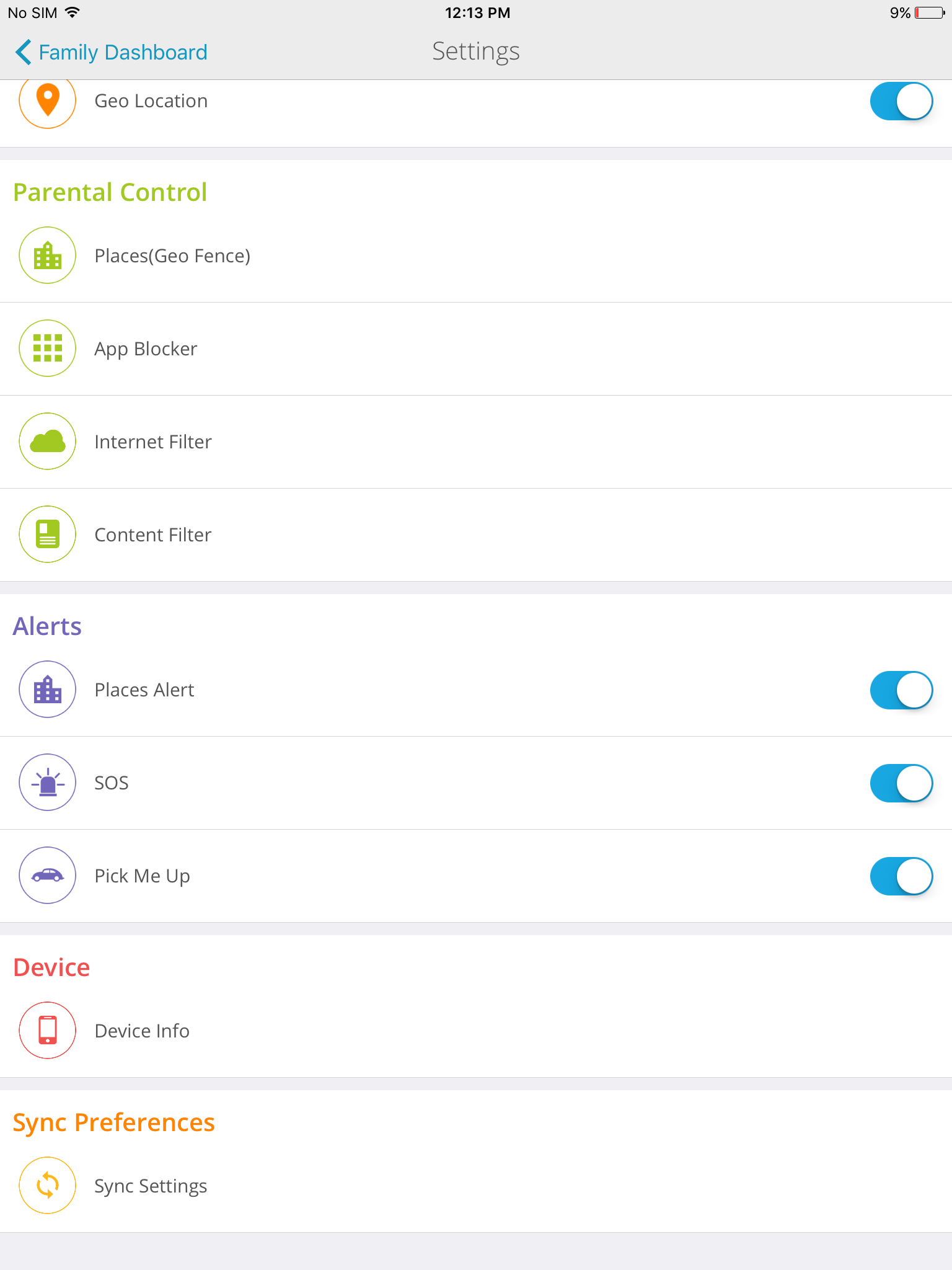The image features a predominantly white background with a gray banner stretched across the top. On the left side of the banner, the text "Family Dashboard" is displayed in blue, accompanied by a left-pointing arrow. Centered within the banner is the time "2:13 p.m." in black, followed by a "settings" icon, while the right side shows a "9% battery" indicator.

Below the banner, the background remains white, presenting what appears to be the layout of a settings menu, organized into several categories, each differentiated by color and separated by narrow gray bars. 

- **Geolocation**: This setting is turned on.
- **Parental Control** (highlighted in green): This category includes options such as Places, Geofence, App Blocker, Internet Filter, and Content Filter.
- **Alerts** (highlighted in blue): This section includes Places Alert (turned on), SOS (turned on), and Pick Me Up (turned on).
- **Device** (highlighted in red): This category features Device Info.
- **Sync Preferences** (highlighted in orange): This section includes Sync Settings.

Each category is distinctly color-coded for easy navigation and quick identification. 

Thank you for watching.